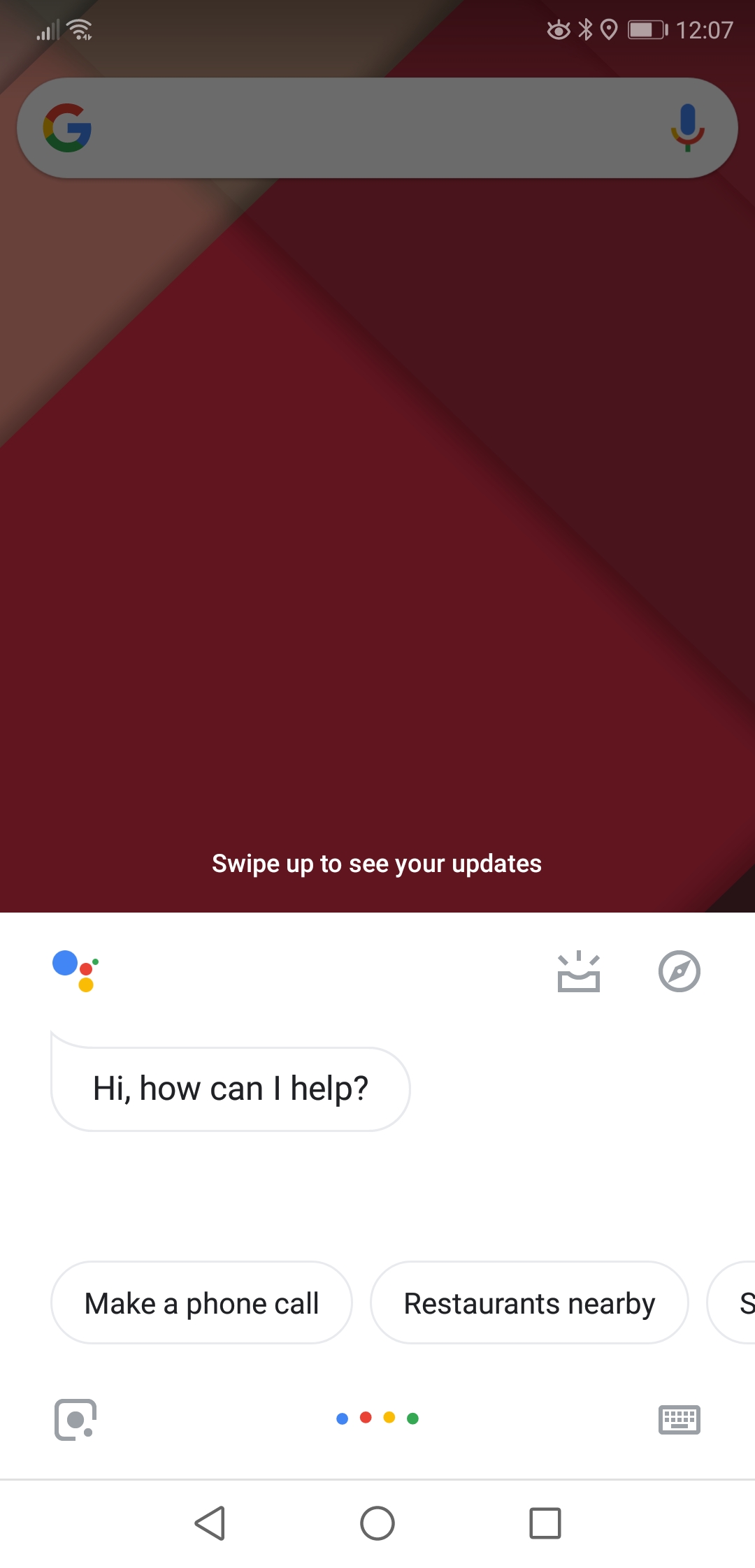A detailed screen capture of a smartphone is displayed, showcasing a chatbot interface prominently. The chatbot greets with, "Hi, how can I help?" and provides options such as "Make a phone call" and "Restaurants nearby," among other unspecified choices. The screen also features a Google search bar, hinting that the user may have initiated the interaction by voice command. A prompt at the bottom instructs, "Swipe up to see your updates." The timestamp on the phone reads 12:07, with the battery level at approximately 80% charged. Additionally, the user is given the alternative to switch to a keyboard input via a dedicated button if they prefer typing over voice commands. At the bottom of the screen, the standard navigation buttons are visible: a triangle (back), a circle (home), and a square (recent apps). The overall setup suggests the user is likely seeking nearby restaurant recommendations.